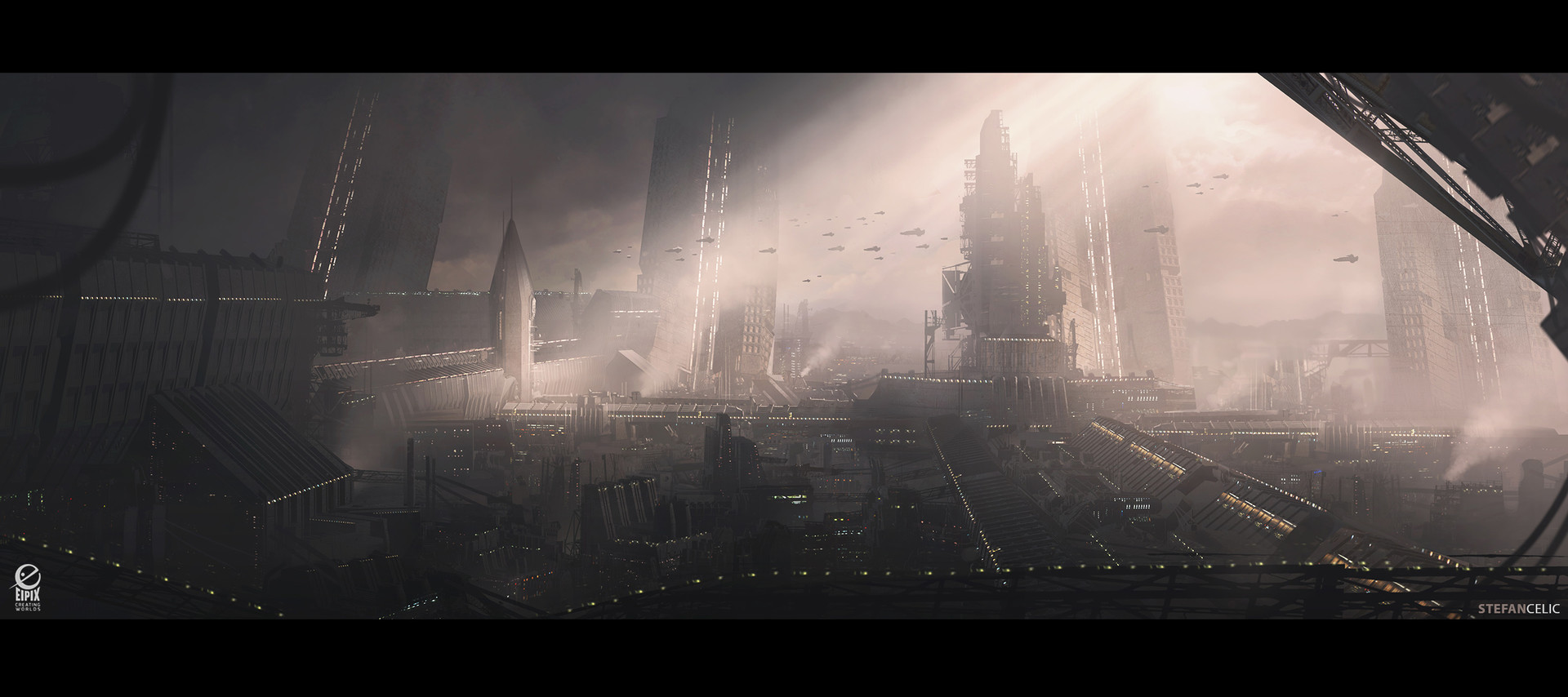The image depicts a surreal, grayscale cityscape bathed in an otherworldly ambiance. Dominated by tall, pointy skyscrapers that rise starkly against a foggy backdrop, the scene exudes an air of mystery and wonder. These towering structures are faintly illuminated by ethereal rays of light cutting through the pervasive darkness, casting a haunting glow over the city. The foreground is framed by unclear objects and shadows, adding to the enigmatic nature of the composition. Scattered throughout the image, especially in the lower sections, are silhouettes and undefined objects, possibly resembling a space station or sci-fi apparatus, suggesting a futuristic setting. The image's overall lack of color, apart from subtle hints of white and yellow light, enhances its noir, unreal quality, making it appear almost like a frame from a dystopian movie or video game. Hidden in one corner is a small, partially obscured logo, hinting that this might be a piece of digital or cinematic art.